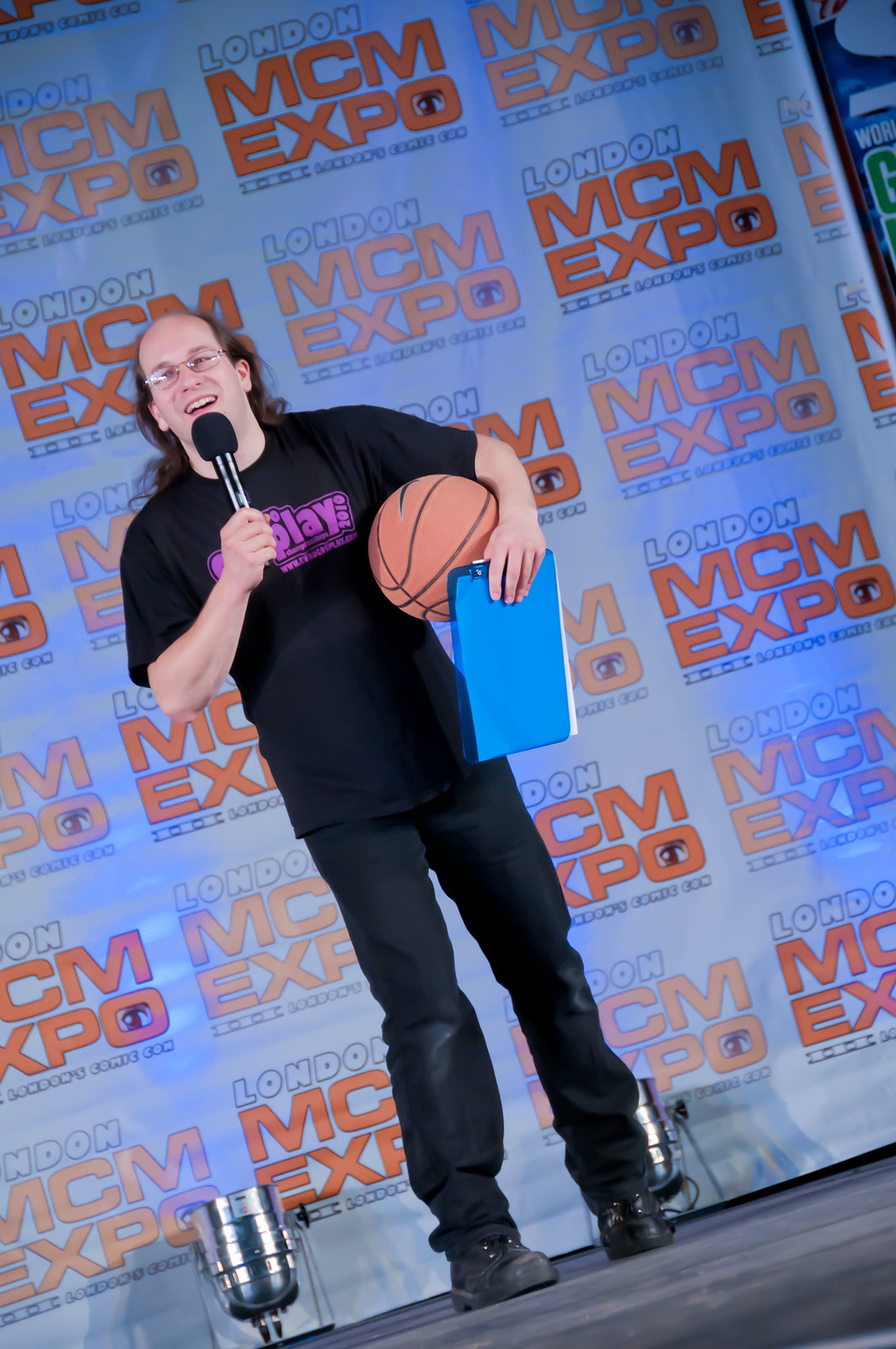A man stands confidently on a dark gray stage, flanked by two large silver spotlights. He is dressed in a black short-sleeved T-shirt, emblazoned with the word "Cosplay," along with black pants and black shoes. The man cradles an orange basketball with black lines in the crook of his left elbow and also holds a clear blue acrylic clipboard with white papers in his left hand. In his right hand, near his face, he grips a black microphone, ready to speak. He wears silver-rimmed glasses and has brown hair, though it appears he might be partially bald. Behind him, the white stage curtain is adorned with a repetitive pattern of orange text that reads "London MCM Expo" and "London Comic Con."